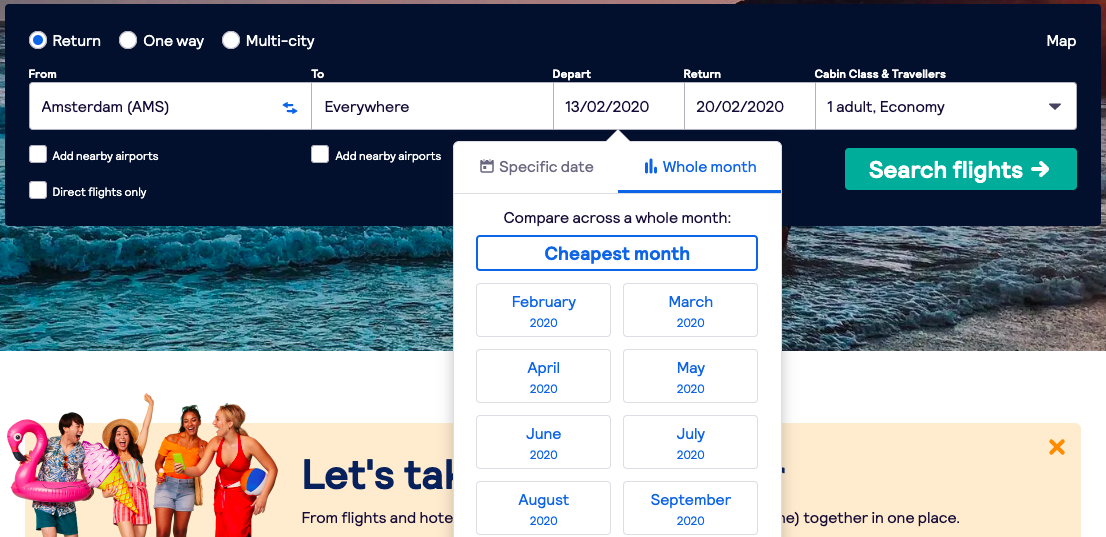Screenshot Description:

This screenshot captures a website interface designed for booking flights. At the top of the screen, a dark navy blue, almost black, horizontal bar spans the width of the page. Along this bar are three small white circles, each accompanied by different option labels. On the upper left-hand corner, there are text options labeled "Return," "One Way," and "Multi-City," with the "Return" option selected.

Directly below the dark bar, a white search form is displayed, featuring specific fields for travel details:
- **From:** Amsterdam (AMS)
- **To:** Everywhere
- **Depart:** 1302 2020 (February 13, 2020)

A drop-down menu expands from the "Depart" field, offering choices to "Specify date" or "Whole month." The user has selected "Whole month," which further provides an option to compare flights across the entire month. Additionally, another selection labeled "Cheapest month" is visible, showcasing month options from February through September within clickable boxes.

- **Return:** 2002 2020 (February 20, 2020)
- **Cabin Class & Travelers:** 1 adult, Economy

Below these fields, a prominent gray rectangle with white text contains a clickable button labeled "Search Flights."

All these elements are overlaid on a background image of waves crashing onto a shore, adding a scenic visual touch to the layout. At the very bottom of the screen, there's a vibrant advertisement banner featuring four people in summer clothing enjoying a party-like atmosphere.

This detailed layout effectively combines practical flight search features with an engaging visual design.